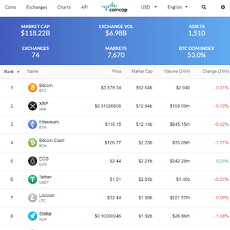This heavily blurred screenshot appears to be taken from an investment assets app. Despite the blurriness, certain details can still be discerned. The app, displayed in English and operating with US dollar currency, showcases a ranking system for various investments, with Bitcoin currently holding the number one spot. A notably long price value is listed next to Bitcoin, accompanied by market cap, volume, and an index, which is likely shown in red to indicate negative growth for Bitcoin. Titles above guide the user through different sections: Market Cap, Exchanges, Markets, BTC, Commerce, Index, Assets, and Exchange Volume. These figures are significant, indicating that the app caters to experienced investors. The interface exhibits a clean, white background with a blue top bar displaying essential statistics.